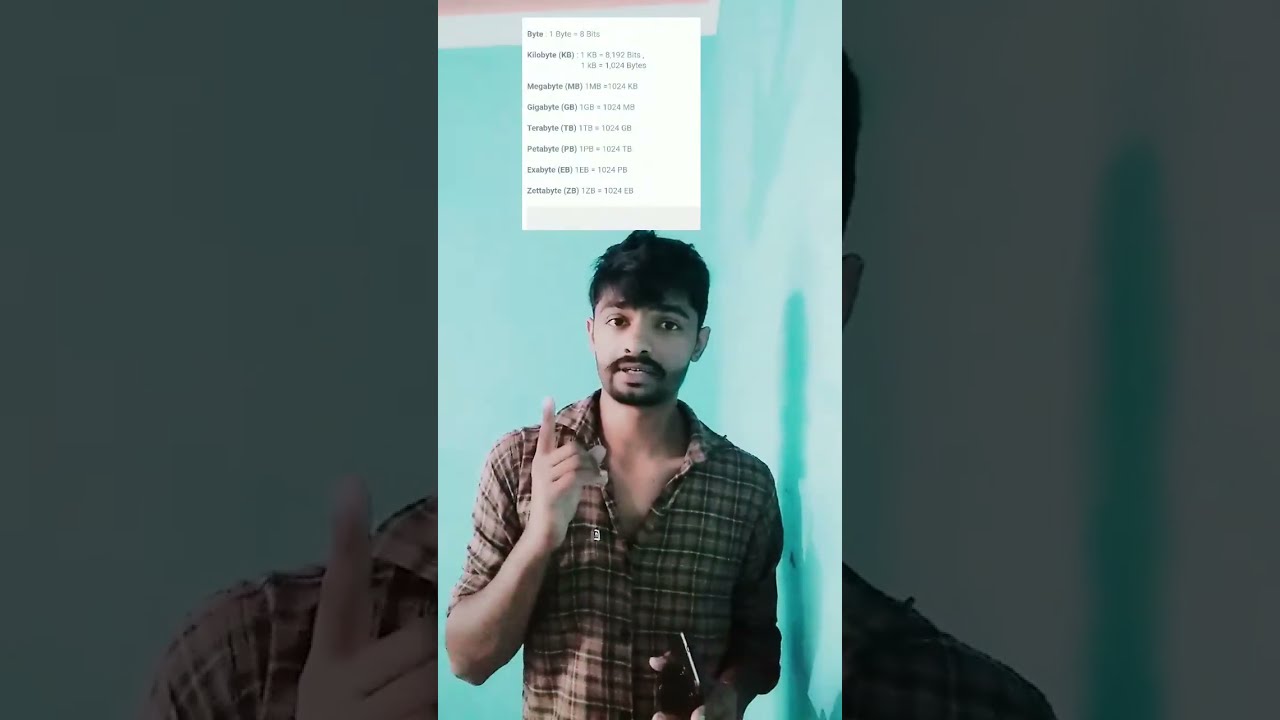The photograph features a man, possibly of Middle Eastern or Indian descent, standing against a backdrop of intersecting light blue and green walls. The walls are adorned with a striped border at the top, boasting white and pink accents. The man has short, somewhat shaggy black hair that falls slightly onto his forehead and thick black eyebrows. He sports a mustache and a closely shaved beard. His attire consists of a brown and medium brown plaid button-up shirt with the top three buttons undone and the sleeves rolled up to his elbows. The man is captured from the waist up, engaging with the viewer through a gesturing pose; his arms are bent at the elbows, extending his hands outward, and he holds a black smartphone in his left hand. The photograph, which is in a portrait orientation, includes substantial white space above his head and is flanked by large black bars on both the left and right sides, each roughly matching the width of the central image.